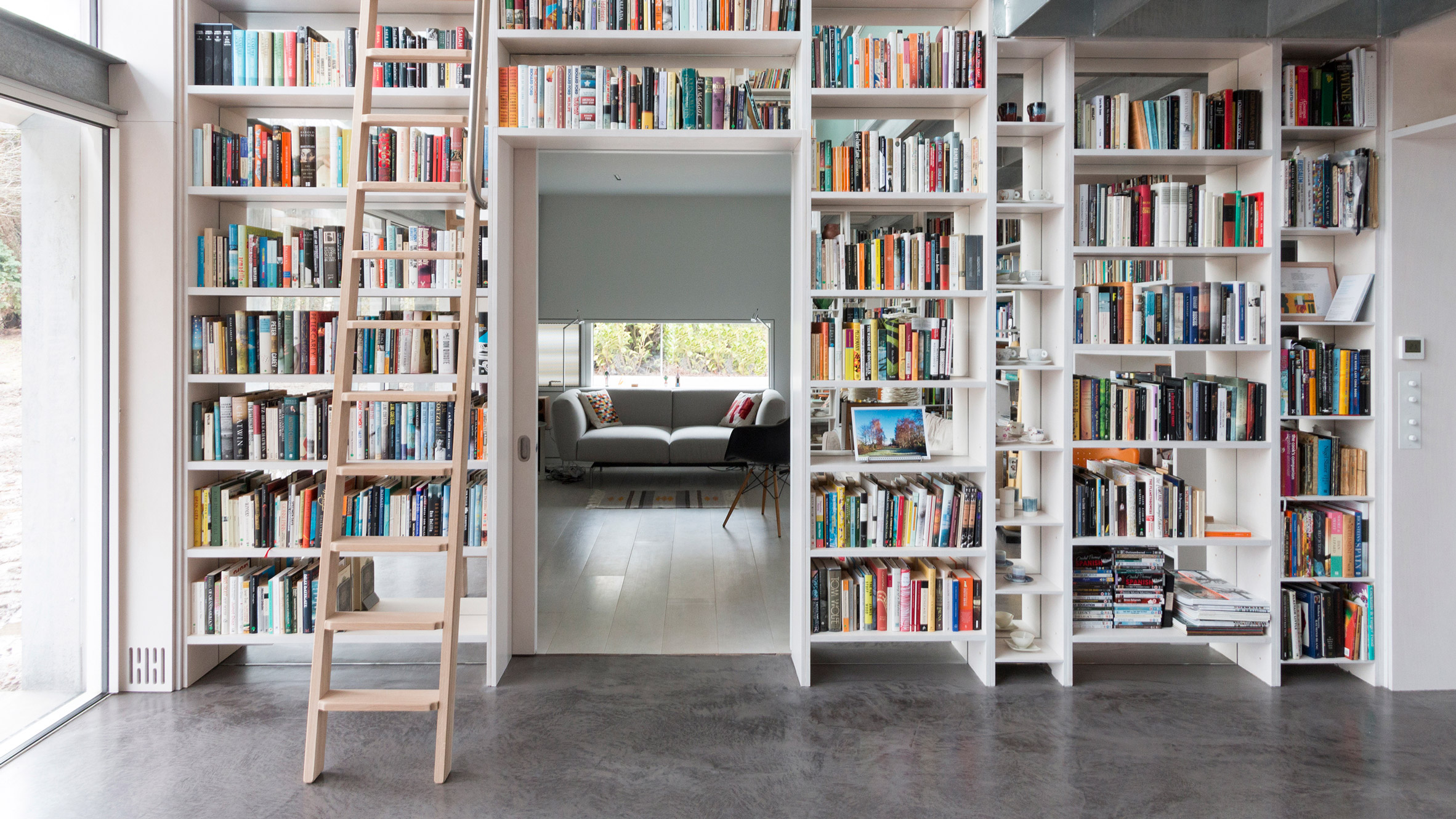The photograph captures an expansive home library with white bookshelves lining the walls from floor to ceiling, stocked neatly with books of various colors including brown, red, yellow, orange, and white. The solid gray concrete floor adds a modern touch to the room. A wooden ladder on the left side of the image hints at the height of the shelves, allowing access to the higher rows of books. A large glass door or window on the left bathes the room in natural sunlight. Through a centrally positioned doorway, a glimpse into a cozy living room reveals a gray couch with two pillows, a black chair, and additional seating, adding a homely atmosphere to the scholarly setting. The overall feel is one of a well-organized and welcoming personal library.